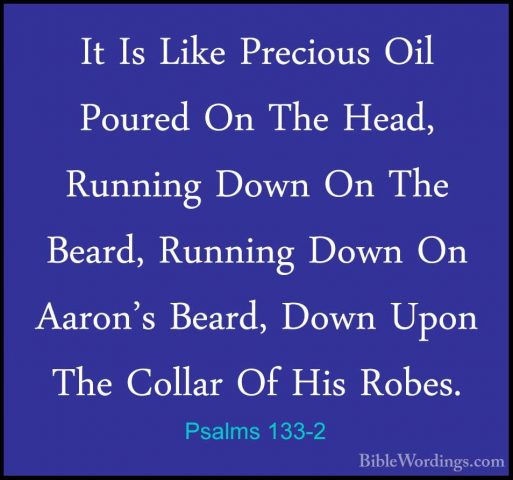The image features a centered biblical quotation displayed on a background with a gradient of dark blue, transitioning to a bright royal blue, bordered by a black edge. The white text reads: "It is like precious oil poured on the head, running down on the beard, running down on Aaron's beard, down upon the collar of his robes." Below this, in turquoise blue, is the citation "Psalms 133:2". In the bottom right corner, the source is noted in purple text as "BibleWordings.com". The simple, religious-themed design and lack of objects or people suggest it could be meant for use in a Bible study setting or by individuals seeking inspiration from scripture.